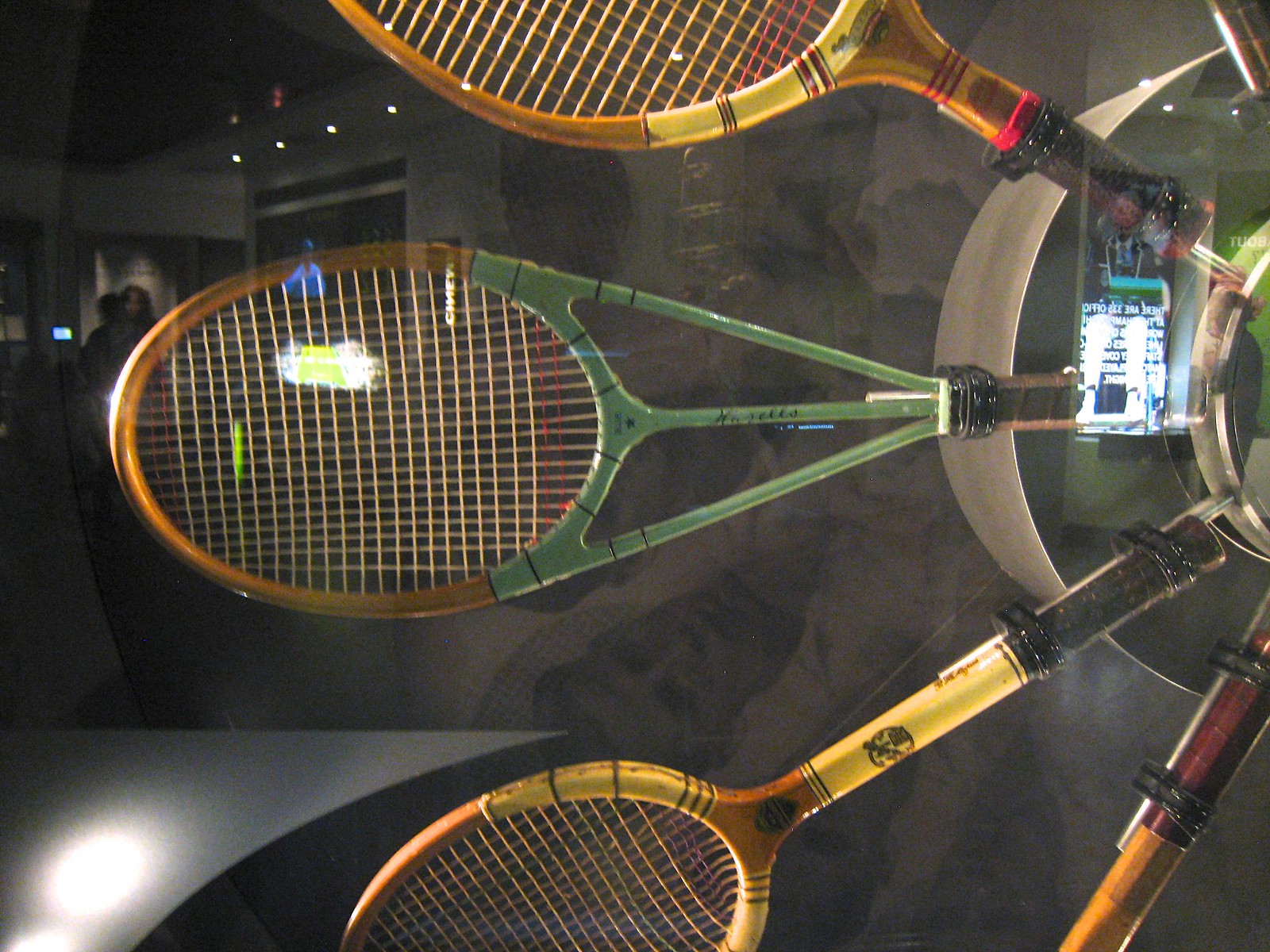The image showcases a striking arrangement of vintage tennis rackets, each with a retro design featuring wooden frames and vibrant colors, reminiscent of the 1970s. The rackets, in shades of green, yellow, and brown, are uniformly attached at their handles to steel rods extending from a central circular metal holder. This setup creates a fan-like display with the racket strings radiating outwards. The background consists of a dark, reflective or smoked glass surface, and faint reflections suggest the presence of a television screen and some indistinct figures and lights behind the camera.